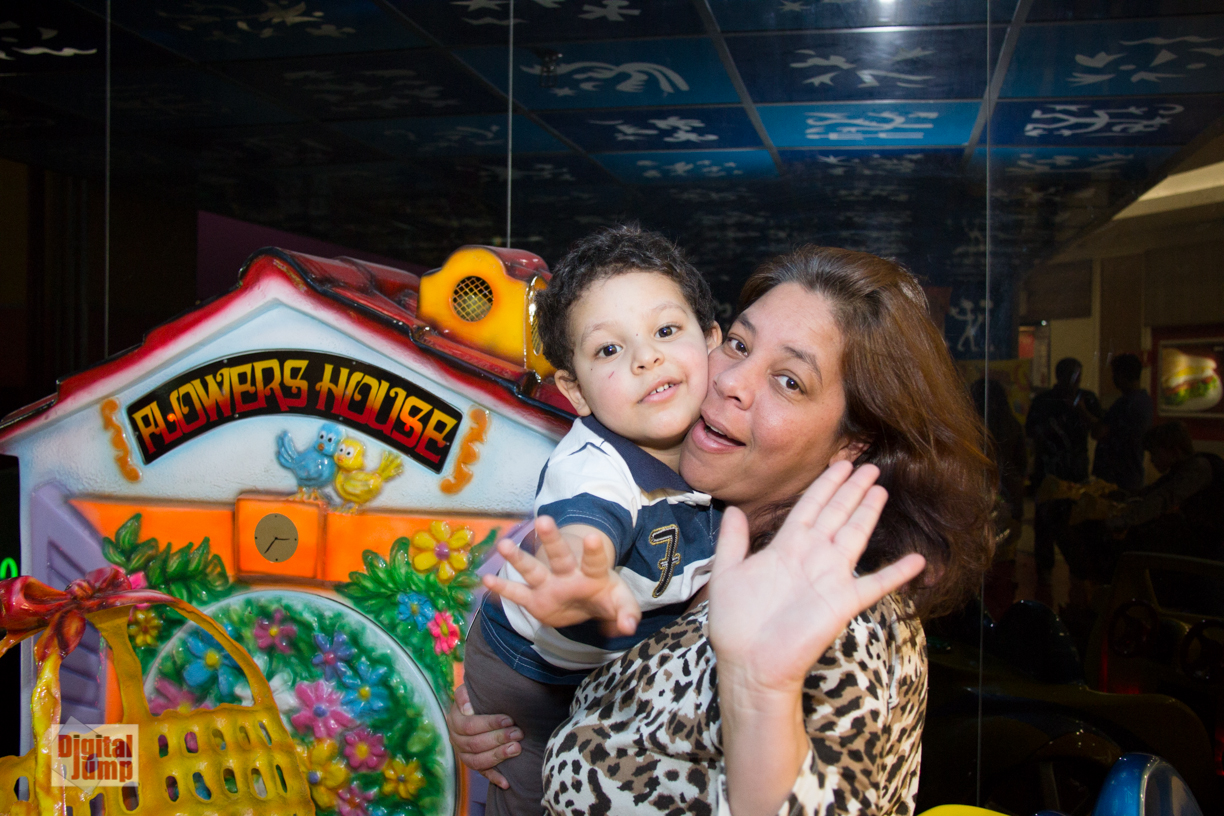In an indoor setting, a woman with brown skin and shoulder-length wavy brown hair, wearing an animal print (leopard) top, is holding a little boy. She's raising her left hand, appearing to wave at the camera, while the boy, with his round face and short dark curly hair, rests his cheek against hers and reaches out his right hand. The boy is dressed in a white and blue striped shirt featuring the number seven and dark-colored trousers. They both seem focused on the camera. Standing next to them is a colorful child’s playhouse with a red roof, yellow features, and the words “Flower's House” written at the top. The playhouse also has decorative elements like leaves, flowers, and illustrations of two birds, one yellow and one blue. The background of the image is quite dim, revealing ceiling tiles with symbols and some indistinct figures standing around. The setup of the scene suggests a lively indoor play area or an amusement zone.